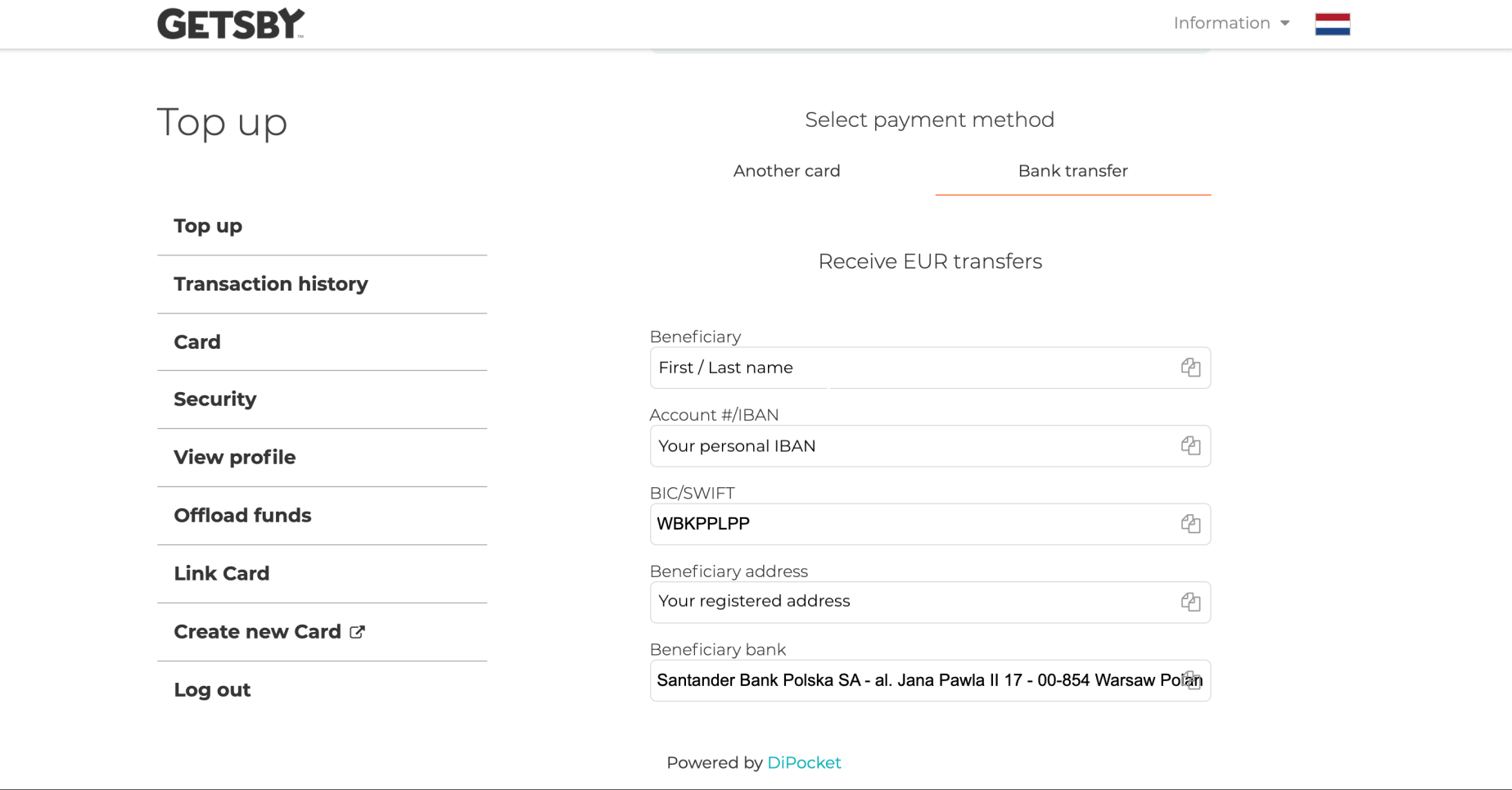This screenshot showcases a web page with a clean white background and a minimalist design. At the very top, there is a header bar featuring "Gatsby" in capital cartoon letters on the upper left corner. On the right side of this header, there is a dropdown menu labeled "Information" and a tri-color flag with red at the top, white in the center, and blue at the bottom.

Immediately below "Gatsby," it reads "Top Up." Along the left side of the page, there is a vertical menu in bold black font listing the following options: Top Up, Transaction History, Card, Security, View Profile, Offload Funds, Link Card, Create New Card, and Log Out. 

On the right side of the page, the top section begins with the heading "Select Payment Method." There are two choices: Another Card or Bank Transfer. The option "Bank Transfer" is underlined with a thin orange line, indicating its selection. Beneath this, the section is titled "Receive EUR Transfers" and features input fields for the following details: Beneficiary (first and last name), Account Number, Your Personal IBAN, BIC/SWIFT, Beneficiary Address, and Beneficiary Bank. The Beneficiary Bank is specified as Santander Bank.

Centered at the bottom of the image, it notes "Powered by DI Pocket," with "DI Pocket" being a clickable blue link. The image has a thin dark line at the very bottom, but no border around the entire image.